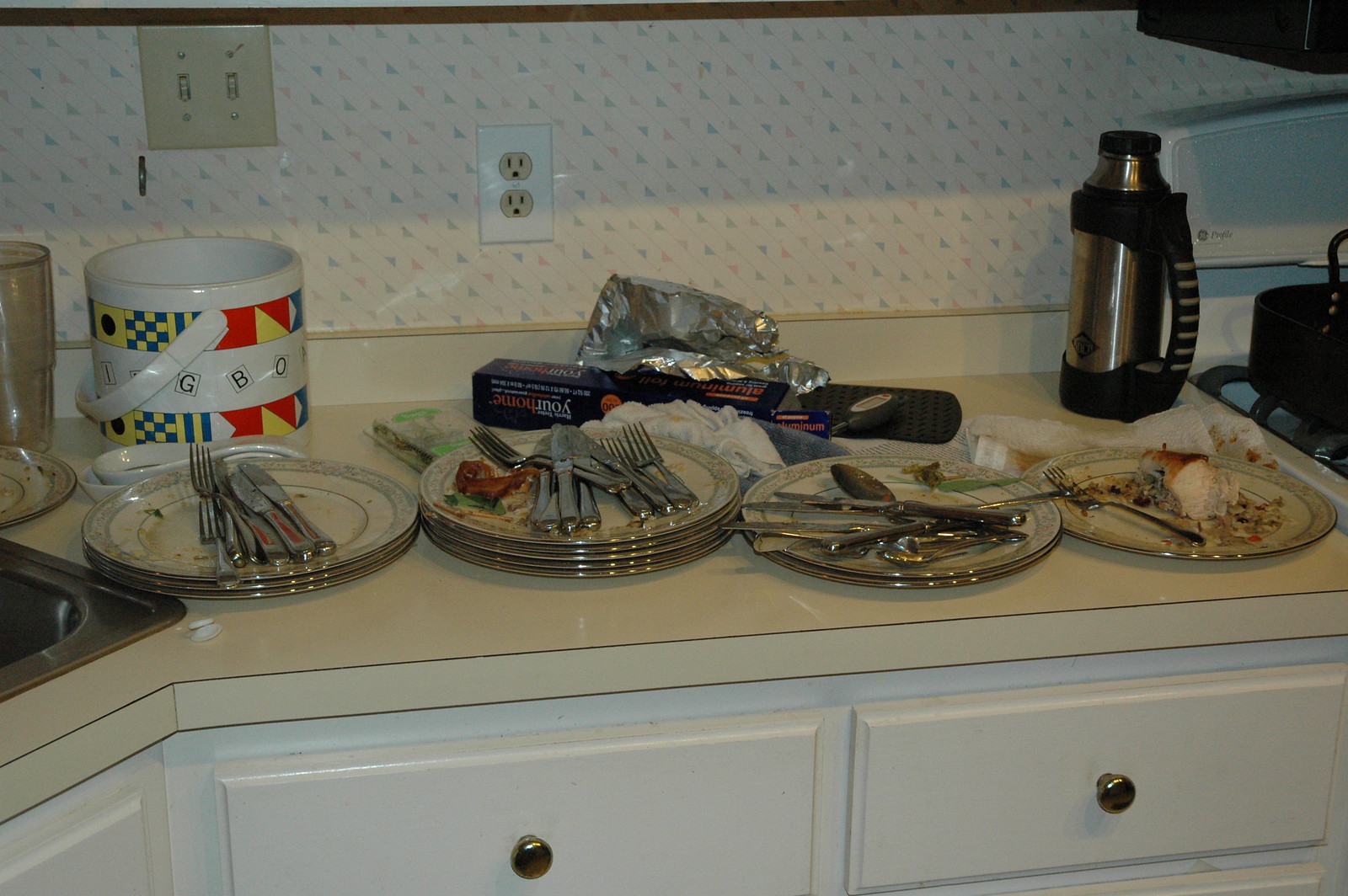The photograph portrays a kitchen counter set against a wall adorned with pinkish wallpaper featuring a pattern of pink, blue, and white arrows pointing in various directions. The countertop itself is a solid yellowish-beige color, possibly linoleum, and is accentuated by a white border where it meets the wall. The wall also includes a white electrical outlet and a dual-option light switch.

Below the countertop, there are white drawers equipped with brass knobs. The counter is occupied by four distinct piles of plates, alongside other items. On the far right, a single plate with leftover food and a fork is positioned. To its left, there is a stack of two plates holding several forks, knives, and spoons. Adjacent to that is another stack, approximately six or seven plates wide, also containing some leftover food and multiple neatly organized forks and knives. The final stack consists of three plates with a few knives and forks arranged on top. 

Behind these stacks, in the background, a cookie jar, a roll of aluminum foil, and a thermos can be seen, completing the scene.